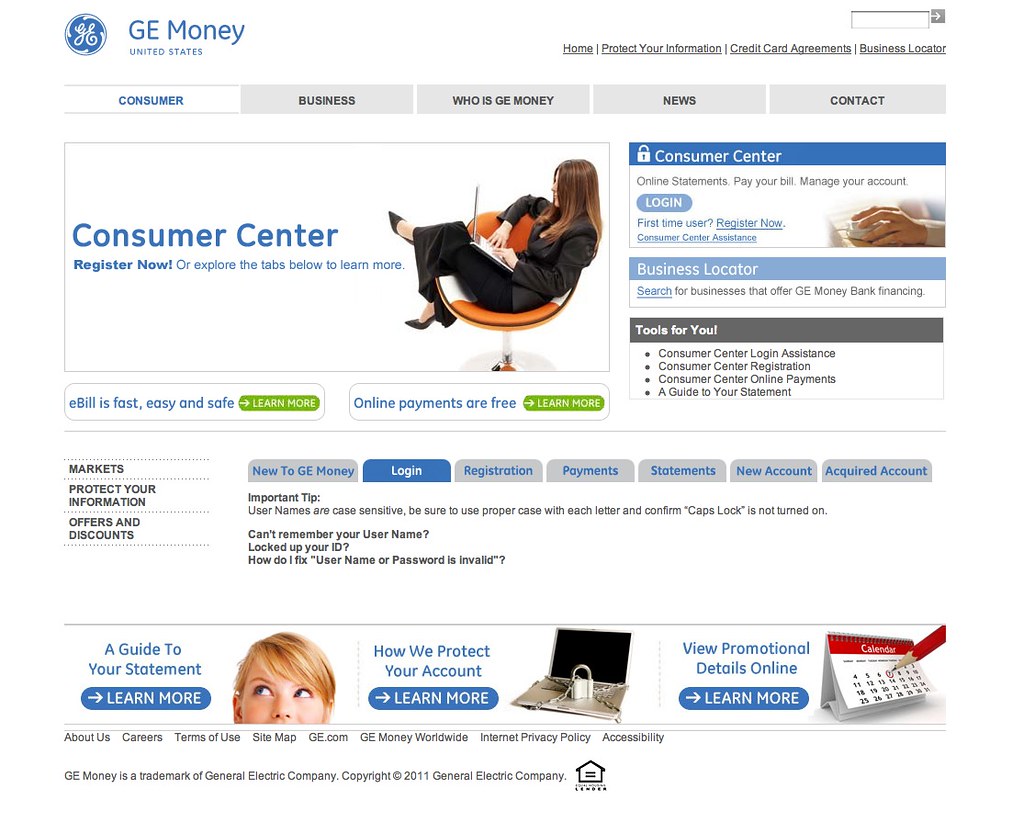This screenshot captures the homepage of a GE Money website. The design features a clean, white background without borders. Prominently displayed in the upper left corner is the GE logo, coupled with the text “GE Money.” Directly underneath, in smaller font, it reads “United States.” 

To the far right, there is a search bar with a grey arrow button, allowing users to input queries. Just below it, there are clickable links, such as "Home," "Protect Your Information," "Credit Card Agreements," and "Business Locator."

The main navigation bar consists of five tabs: "Consumer," "Business," "Who is GE Money," "News," and "Contact." The "Consumer" tab is highlighted in white, indicating it is the selected page, while the others remain in grey. 

The body of the webpage is divided into several sections. On the left, there's an image of a woman seated in a chair next to headers like "Consumer Center" and "Register Now." Adjacent to this, more consumer-related options are displayed, including login portals and various tools.

Further down, there are numerous clickable links tailored for different user needs such as market information and account protection. This section also includes tabs for features like "New GE" and "Log In," with "Log In" being the currently selected tab.

At the bottom of the page, three distinct sections are presented side by side: 

1. "A Guide to Your Statement" featuring an image of a woman looking up.
2. "How We Protect Your Account" with a "Learn More" button.
3. "View Promotional Details Online," also accompanied by a "Learn More" button.

Each section is designed to provide users with additional information and resources, enhancing the overall user experience.